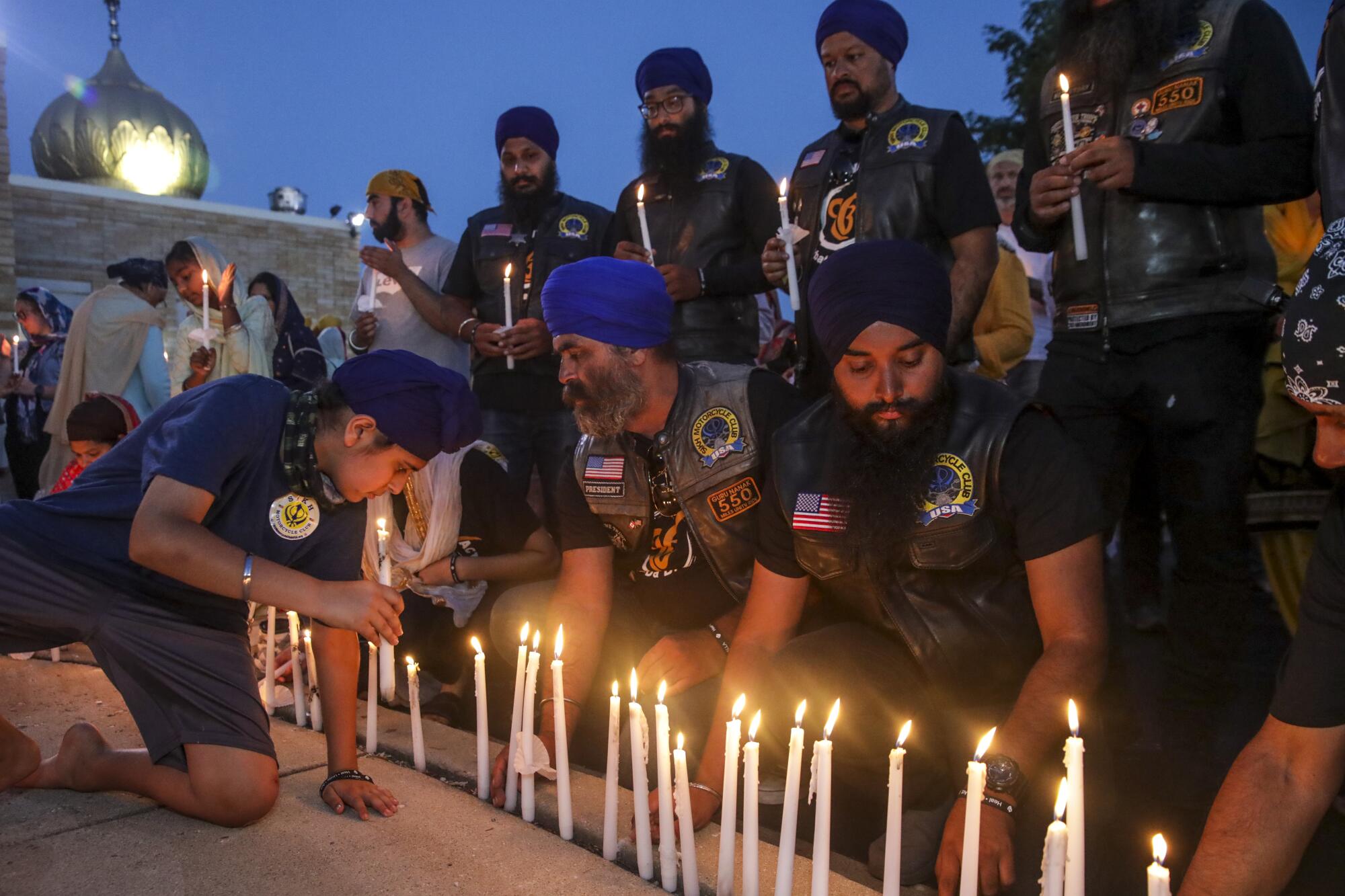The image captures a serene outdoor scene at dusk, where a group of men, each wearing head coverings like turbans, are engaged in a ritualistic candle-lighting ceremony. In the foreground, a man is kneeling, tending to a line of long, thin white candles that are placed on the ground, all lit and spreading a gentle glow. Behind him, a row of men is also kneeling, their attention focused on the candles. Standing behind these kneeling men is another row of men, each holding a lit candle. 

In the middle of the picture, closer to the left side, a woman is also kneeling near a candle, her face softly illuminated by its light. The participants seem to be preparing or engaging in prayer or a cultural observance, indicated by their ritualistic movements and the reverence in their postures. 

The background reveals a building with an interesting top, featuring a large dome that suggests a style foreign to the U.S., perhaps Arab or Middle Eastern. Despite the falling darkness, the clarity of the image allows for detailed observation of the participants and their solemn activities, creating an atmosphere of tranquil devotion.